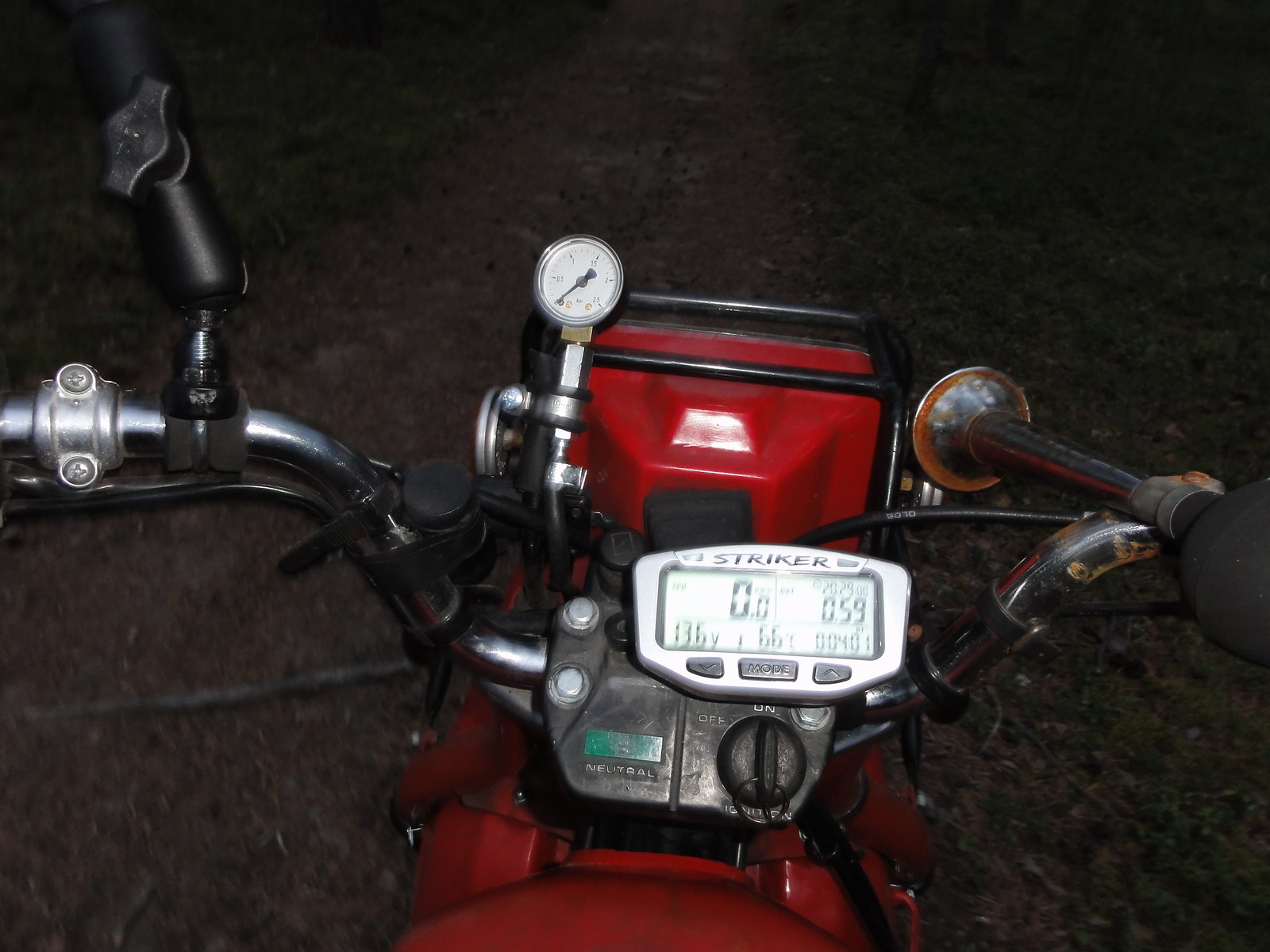In the image, a striking red motorcycle, possibly a scooter, stands prominently against a shadowy and rugged background, suggesting it might be parked on the floor of a garage or a road. The motorcycle is illuminated, highlighting its chrome-plated handlebars and black brake cables. On the right-hand handlebar, there is an upright structure with an adjustable device whose purpose is unclear. On the left-hand side, a gauge, possibly but doubtfully a speedometer, extends upwards. The centerpiece of the handlebars features a silver plate with the name "Stryker" emblazoned on it, displaying four distinct gauges that start at zero, and two smaller indicators nestled underneath. The same plate also has a fuel filler cap. To the left of this setup, a green label is visible, though its text is not legible. Additionally, a sizable horn with an open end and a bulb attached serves as a warning device. The red paint of the motorcycle, which appears slightly oily, adds to its eye-catching appeal.